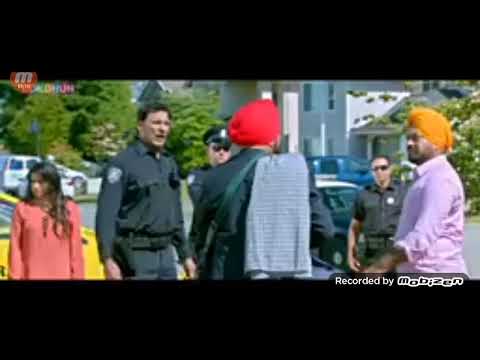The image, possibly a video snapshot, features black borders at the top and bottom, creating a 16:9 aspect ratio. At the center, a man with his back to the camera wears a red turban and a black top with blue fabric draped over his right shoulder. He is facing a police officer clad in uniform with dark sunglasses and a hat. To the right of the central figure stands another man in a pink shirt and orange turban. Approaching these two men are three distinct police officers. On the left third of the image, another officer, identified by a shield on his right shoulder patch, is engaged in conversation. A girl with long, brown hair and an orange shirt is positioned nearby. The scene is set outdoors in a residential neighborhood, discernible by the visible vehicles, houses, trees, large flower bushes, and a porch. The text "Recorded by Moby Zinn" appears at the bottom right corner of the image.